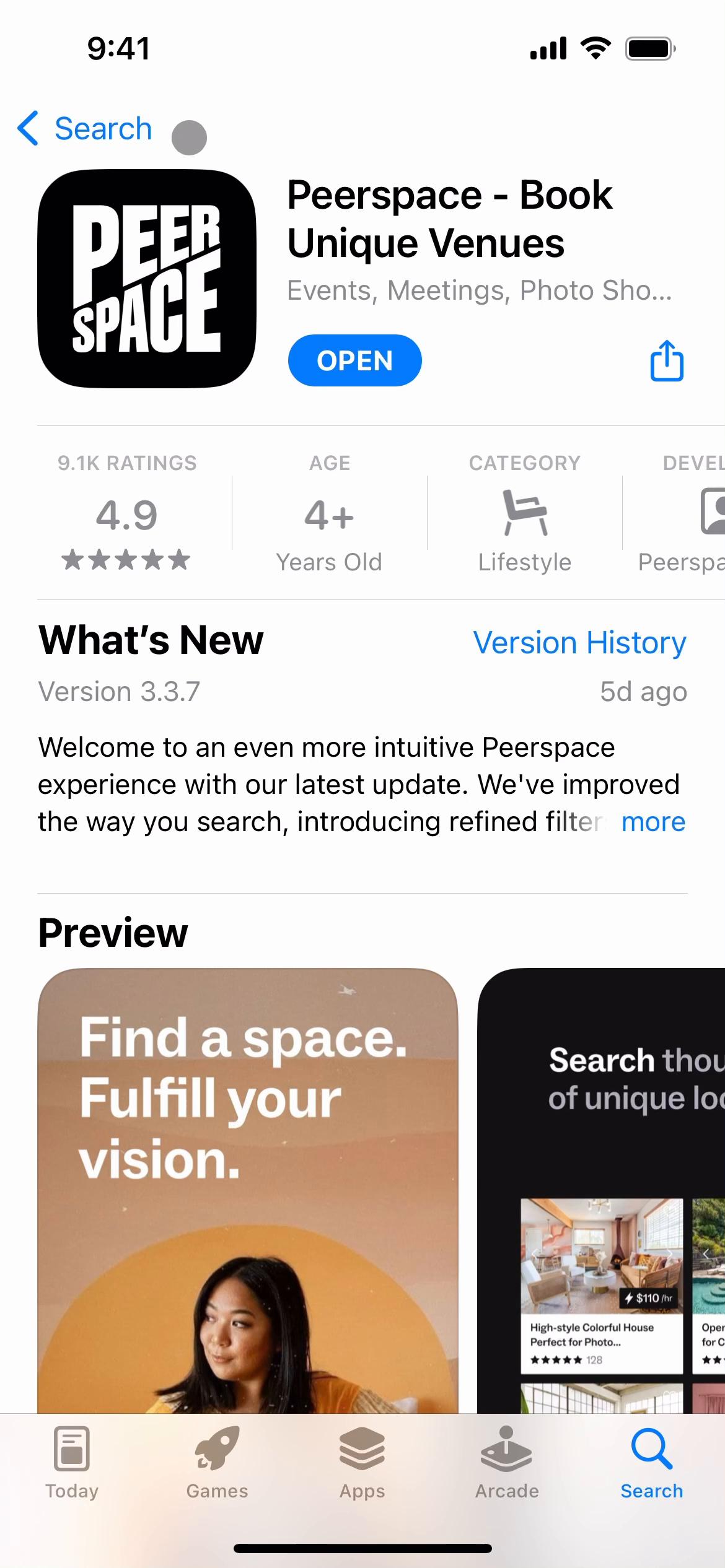Sure, here is the cleaned-up and detailed caption:

---

This image is a screenshot of the mobile app 'PeerSpace' displayed on a smartphone. 

The screenshot was taken at 09:41, as shown by the time at the top left corner of the screen. The phone's status bar indicates a nearly full battery and an active Wi-Fi connection.

The app interface is set against a white background and features a black square with rounded edges at the center. Inside the black square, the text "PeerSpace" is displayed in capital white letters, arranged diagonally. Beneath this, it reads "Book unique venues for events, meetings, photoshoots..." 

There's a prominent blue button labeled "Open." Below this button, user feedback is showcased: "9.1K ratings," an impressive "4.9 out of 5 stars," and the age rating "4+ years old." The app falls under the "Lifestyle" category, represented by a small icon of a chair.

Further down, a section titled "What's New?" is presented in black text. The version "3.3.7" update notes mention improvements for a more intuitive PeerSpace experience, including refined search filters. The version history indicates that this update was released five days ago.

The screenshot also includes an advertisement featuring a Southeast Asian woman with black hair, looking to her left. She is seated in front of a wall adorned with a design resembling a yellow sun with sunset hues fading upwards. Overlaying this image, white text reads: "Find a space. Fulfill your vision."

At the bottom of the screen, icons for "Today," "Games," etc. are faintly visible.

---

This updated caption should provide a comprehensive and detailed description of the image in question.